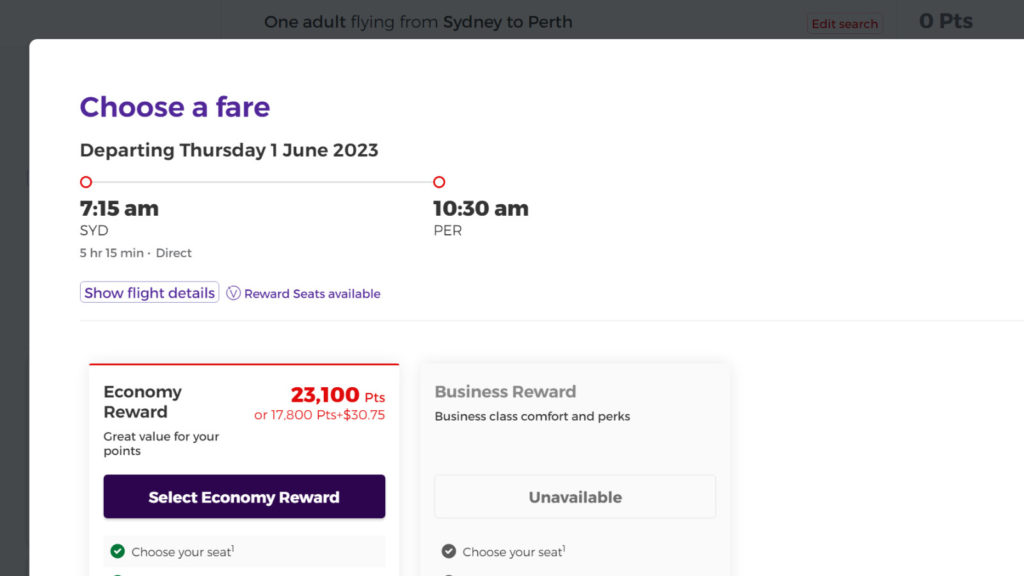This landscape-oriented screenshot captures a travel planning website interface, predominantly displaying a white screen with a grayed-out background on the left and top sections. At the top left corner of the central white section, the words "Jews Affair" appear in purple font, accompanied by "Departing 1 June 2023" in black font right beneath it.

Central to the image are two orange circles connected by a horizontal line. On the left circle, it indicates a 7:15 AM departure from SYD, detailing a direct flight duration of 5 hours and 15 minutes. The right circle marks the 10:30 AM arrival in PER. Beneath this timeline, a purple button prompts "Show Flight Details," while a second purple button indicates "Reward Seats Available."

Separated by a thin gray line, the lower part of the screen features two distinct boxes on the left. The first box is white, rectangular, slightly longer than tall, and edged with a red border at the top. Inside, the text reads "Economy Reward, great value for your points" on the left, with a cost of "23,100 points or 17,800 points + $30.75" in red on the right. A purple button below allows users to "Select Economy Reward."

To the right is a grayed-out box labeled "Business Reward, Business Class Comfort and Perks," above an "Unavailable" rectangular notification. At the bottom, a gray check mark indicates the option to "Choose Your Seat."